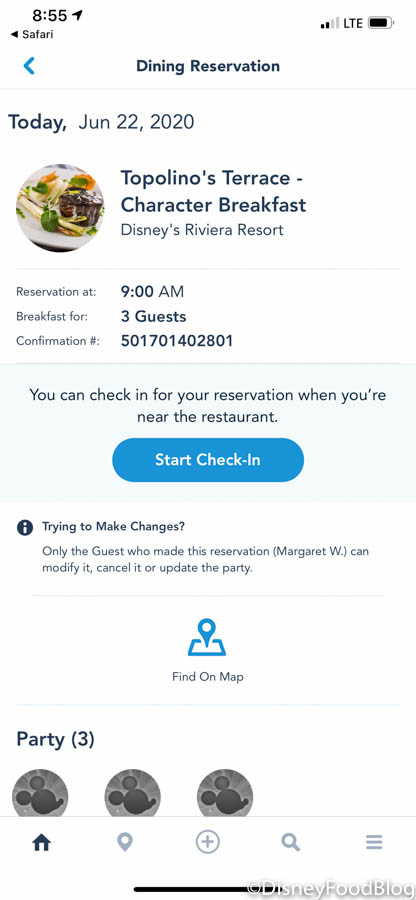The image portrays a detailed snapshot of a phone screen displaying a dining reservation confirmation. The phone, operating on LTE with a full battery, shows the time as 8:55 AM and indicates the Safari browser is in use. The screen displays a reservation for Topolino's Terrace Character Breakfast at Disney's Riviera Resort, dated today, June 22nd, 2020.

Prominently featured is a circular image of an elegant dish adorned with vibrant green leaves, hints of orange, and brown hues, hinting at the gourmet nature of the food. Below the image, it specifies that the reservation is for 9 AM for three guests. 

A confirmation number is shown, followed by a note indicating that check-in can be done when near the restaurant. There is a blue "Start Check-In" button just below this note. Only Margaret W., the individual who made the reservation, has the capability to modify, cancel, or update the reservation through a "Make Changes" option. Additionally, there’s a “Find on Map” feature indicated by a blue icon of a person.

Three black-and-white Mickey Mouse icons are visible, representing the three guests. At the bottom of the screen, there are clickable phone and map icons, and the webpage is attributed to Disney Food Blog.